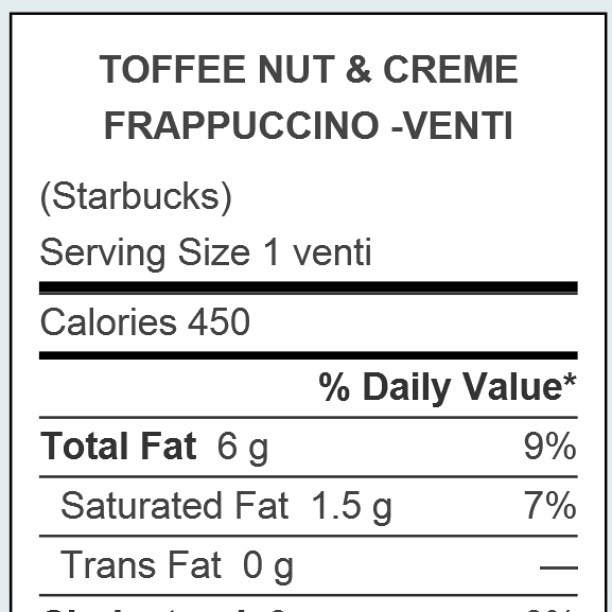This image features the Nutrition Facts label of a Starbucks Toffee Nut and Cream Frappuccino in a Venti size. The label is predominately black-and-white, with "Toffee Nut and Cream Frappuccino Venti" written at the top. The term "Starbucks" is enclosed in parentheses next to it. Below this heading, it lists a serving size of 120. The label provides detailed nutritional information, including the number of calories, and the percentage of daily values for fat, saturated fat, and trans fat. Due to some words being cut off at the very bottom of the image, the full nutrition information cannot be seen. A slight gray border wraps around the Nutrition Facts box, giving it a defined outline.